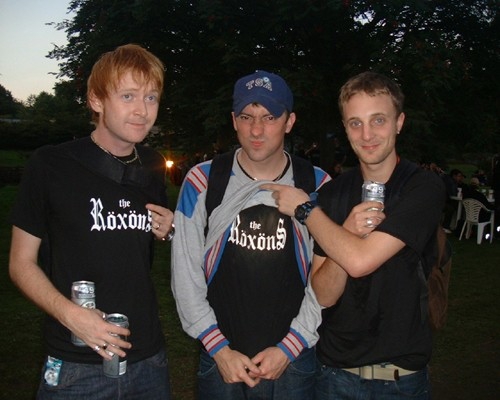The outdoor photograph, taken at dusk, captures three young men posing together. All three are wearing blue jeans and black T-shirts bearing the logo "The Roxsons." The tallest on the left, a white man with long red hair, is looking away from the camera while holding two beer cans—one against his stomach and the other in his hand. In the middle, a young man with a grey sweater over his T-shirt and a blue baseball cap with "TSA" on it is making a duck face. His friend on the right, a white man with short blonde hair wearing a black watch, is lifting the middle man's sweater to reveal the Roxsons logo on his T-shirt, while also holding a beer can. In the background, amidst the darkening sky, several plastic chairs and trees are visible with a few people seated.